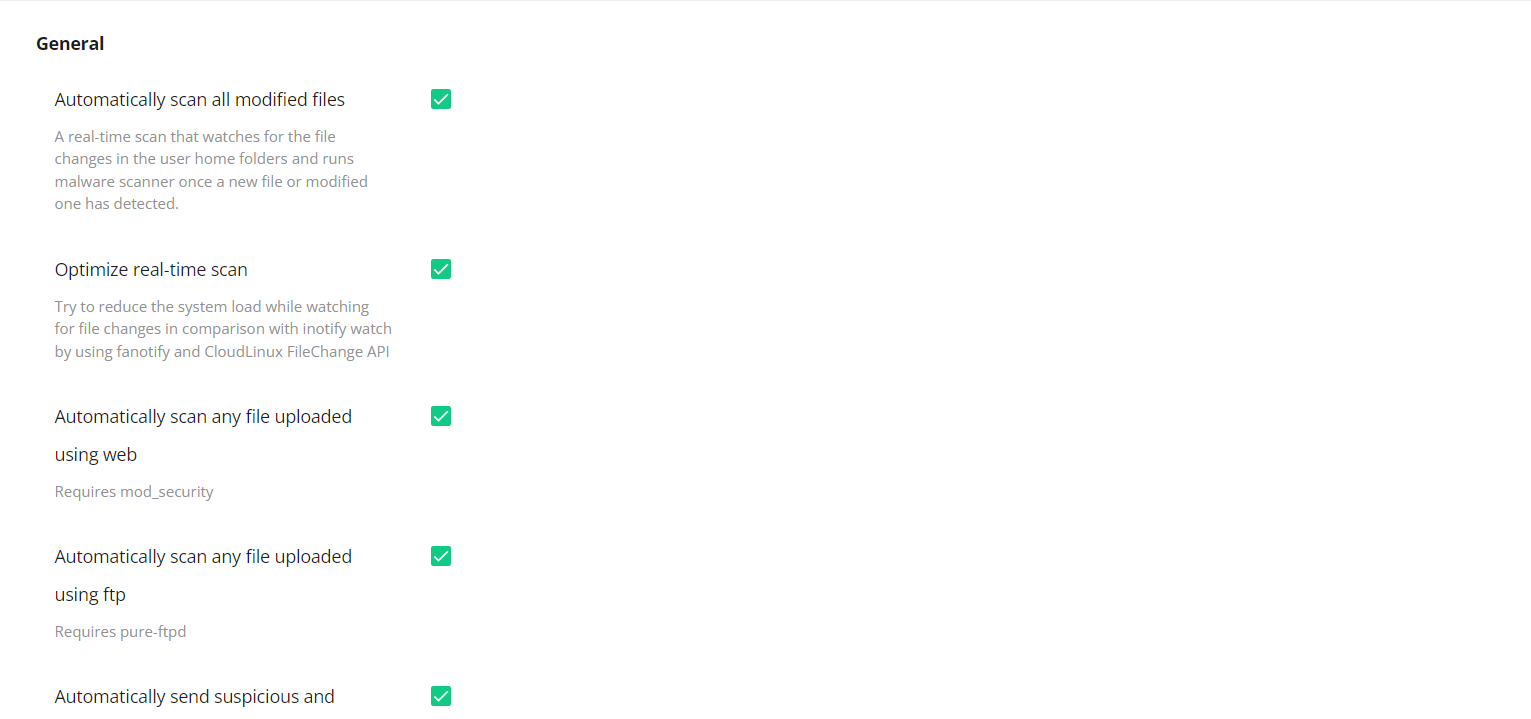This image depicts the settings section of a web interface or a mobile application. The interface appears streamlined, with the content aligned to the right side. Only one visible border is present at the top as a horizontal line stretching across the width. The majority of the image is predominantly blank, occupying over two-thirds of the space, leaving the settings content compacted into the remaining third.

At the top of the visible content, the word "General" is displayed in bold, aligned to the left within the title area of the screen. Directly below this, a subheading states, "Automatically scan all modified files", accompanied by a green checkbox to the right that indicates this option is enabled.

Following this, a paragraph explains that a real-time scan monitors changes within the user's home folders to run a malware scan whenever new or modified files are detected. Below this explanation, another setting labeled "Optimize real-time scan" is shown.

A subsequent paragraph suggests the purpose of this feature is to minimize system load while tracking file changes. The text likely continues to provide further details, although part of the description remains unreadable due to distance.

Further down, additional options appear: "Automatically scan any file upload using web", "Automatically scan any file upload using FTP", and "Automatically send suspicious..." The text cuts off here, indicating there might be more information related to suspicious file actions.